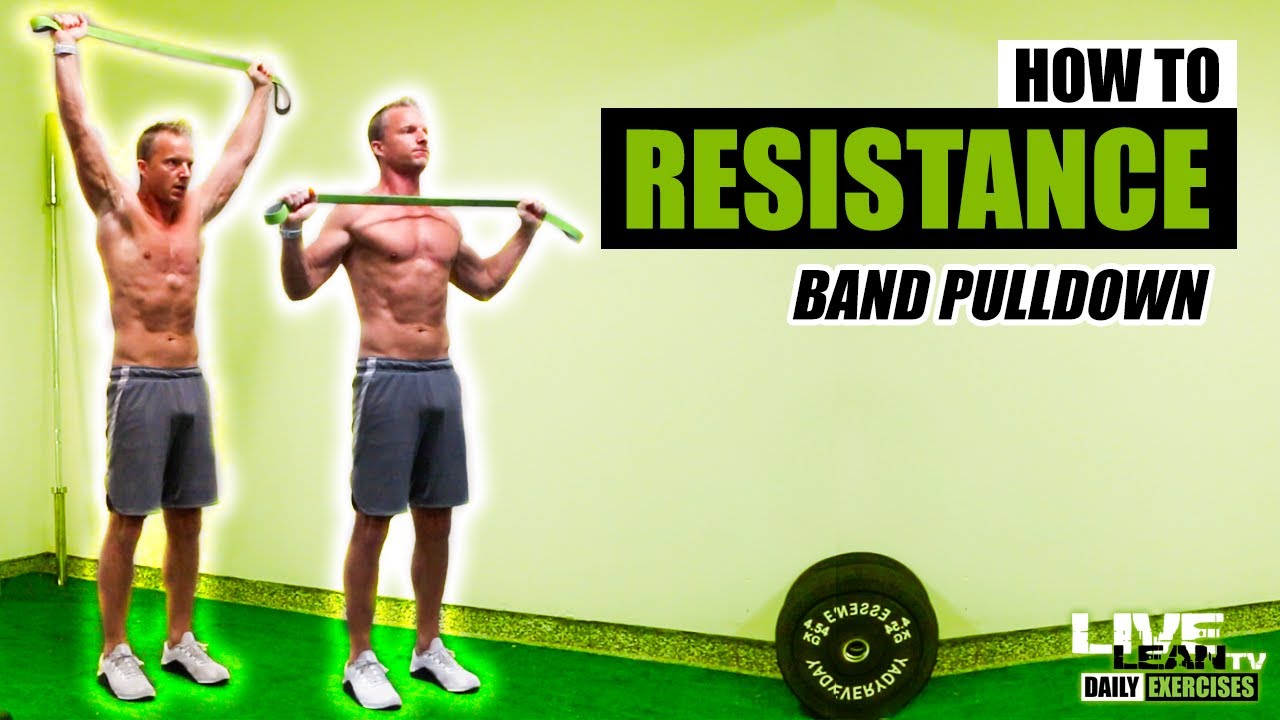This image, likely from an exercise website, features two side-by-side photos of the same man demonstrating a resistance band exercise against a light yellowish-green wall that becomes more colorful toward the left. The man, a white trainer with short blonde hair, is shown twice. In the left image, he is standing on a neon green carpet, holding a green resistance band directly over his head with both hands. In the right image, he holds the band near his shoulder level. He is wearing gray shorts that reach his knees and white sneakers with black soles. Both pictures show him looking to the left. The text on the image reads "How to Resistance Band Pull Down," with the words "How to" in black letters on a white background, "Resistance" in green letters on a black background, and "Band Pull Down" in black letters again on a white background. Below the images, black weights are visible leaning against the wall. In the bottom right corner, the logo "Live Lean TV Daily Exercises" is displayed.